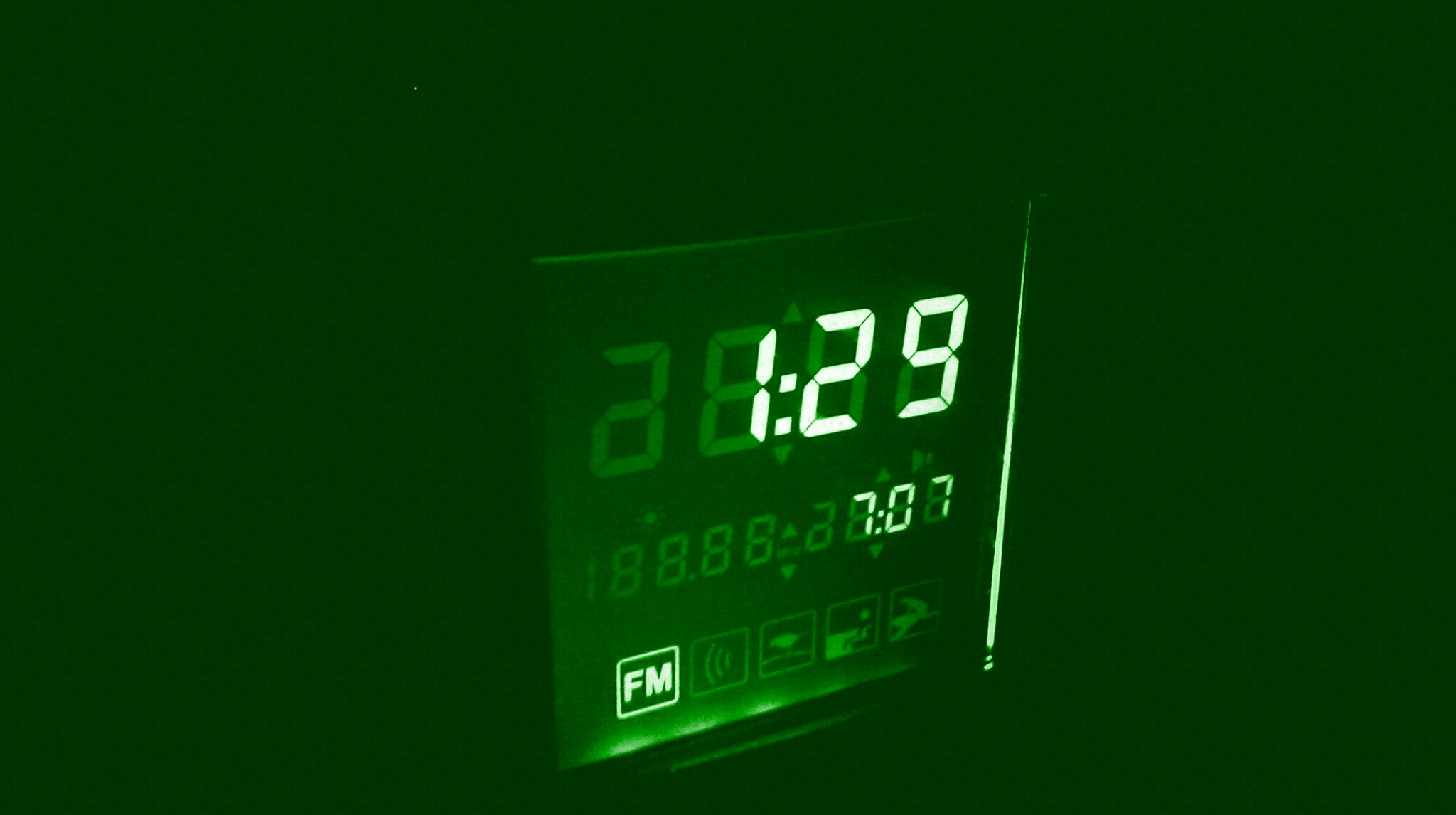The image depicts a digital display with a predominantly dark green background. The display screen itself is a darker shade of green, featuring very light green, almost white, numerals. At the top of the screen, the large numbers "1:29" are displayed, likely indicating the current time. Below this, in smaller text, the numbers "7:07" are visible, whose purpose remains unclear. Beneath these numbers, a series of icons are present, with the first box on the left illuminated and displaying "FM," likely referring to an FM radio function. The adjacent icons include a Wi-Fi symbol and three other shapes resembling a bird, a cliff, and a cat standing on a car, although their exact meanings are uncertain. The display is surrounded by a mostly dark environment, possibly hinting at a night setting, leading to the assumption that this could be part of a car’s center console or a clock radio.